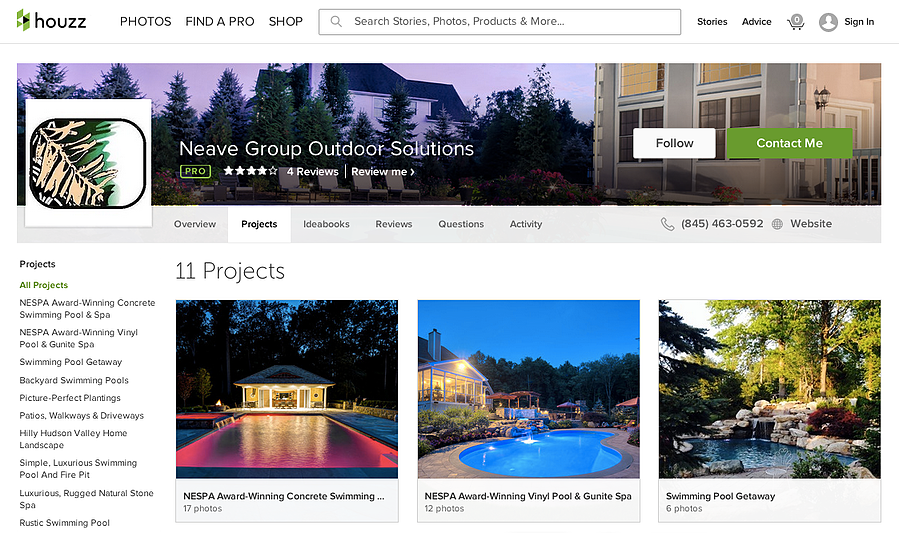This is a detailed screenshot from the search page of Houzz, a real estate website prominently showcasing its name and logo on the top left side of the header. The header also features a comprehensive menu bar, including categories such as Photos, Find a Pro, and Shop, all aligned on the same row as the logo. Adjacent to the Shop link on the right, there's a search bar, followed by four additional icons and links. The first two are text links titled Stories and Advice. The subsequent icons include a shopping cart marked with a zero and a sign-in option represented by a silhouette avatar.

A top banner showcases a profile for Neve Group Outdoor Solutions, displaying a serene mountain resort as the background imagery. This banner includes interactive elements such as a Follow button (white) and a Contact Me button (green), along with the Neve Group's logo on the far left. This profile has garnered four views and boasts a four-star rating.

The page highlights 11 distinct projects with thumbnail images for three of them. The first project features a NESPA award-winning concrete swimming pool with 17 accompanying photos. The second project showcases a NESPA award-winning vinyl pool and Goodnight Spa, consisting of 12 photographs. The third project, titled "Swimming Pool Gateway," includes six photos. 

A sidebar titled "Projects" lists an array of detailed project types, ranging from NESPA award-winning concrete swimming pools to rustic swimming pools, indicating the variety and quality of work showcased by the Neve Group.